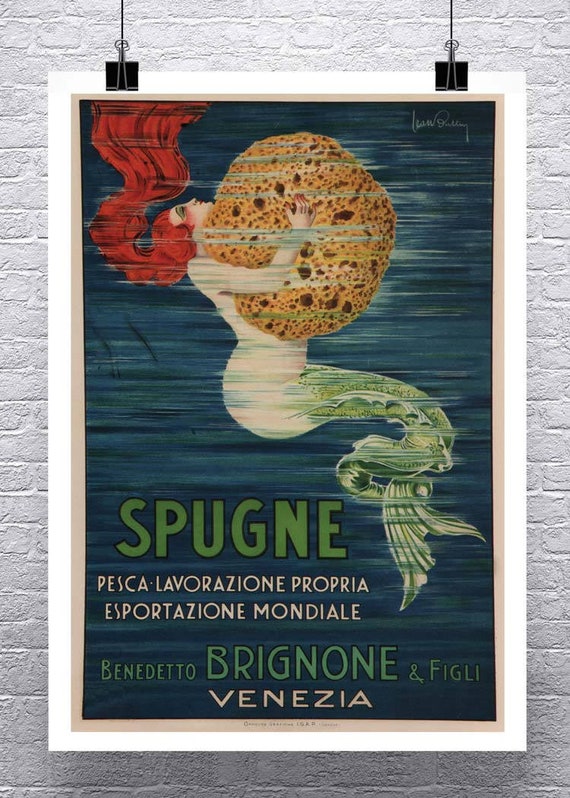This image features a detailed painting displayed against a white brick wall, held up by two heavy-duty black paperclips with visible suspension wires. The painting, mounted with a white border followed by a beige border, depicts an underwater scene with a striking mermaid as its focal point. The mermaid, possessing long, wavy red hair and adorned with green eyeshadow and red lipstick, is depicted with a light green fish tail. In her right arm, she clutches a large, orange porous sponge the size of her body. The water surrounding her is painted in various shades of blue and green to convey depth and movement.

At the bottom left of the painting, the word "SPUGNE" is prominently displayed in green letters, signifying the sponge she holds. Beneath it, in white letters, are the words "PESCA LA LAVORAZIONE PROPRIA ESPORTAZIONE MONDIALE," followed by "BENEDETTO BRIGNONE E FIGLI" in green, and finally, "VENEZIA" in white. The top right corner of the painting bears a signature in white cursive, although it is not legible. The lighting in the room highlights the texture of the brick wall, adding to the display's overall ambiance.